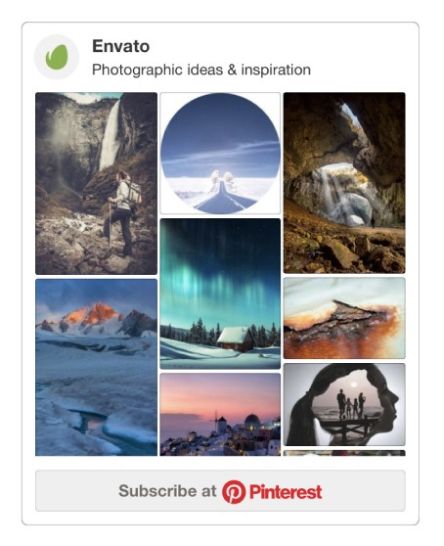The image appears to be a screen capture featuring a promotional banner from Envato, specifically titled "Photographic Ideas and Inspiration." The banner is enclosed within a white box with a thin gray border. At the top of the banner, the word "Envato" is displayed in bold black letters, accompanied by a gray-white circle containing a green leaf icon.

Below the header, a series of photographic thumbnails are arranged in a visually engaging manner. There are a total of seven clearly visible images, with an eighth one partially seen at the bottom.

1. The first image depicts a person dressed in a light-colored sweatshirt or hoodie and dark pants, hiking through a rocky terrain. They carry a hiking stick and wear a backpack. The scenery includes gray rocks, green moss, a waterfall, and a view of the sky.

2. Directly below, the second image captures an arctic tundra landscape. It features ice, a small body of water, a snowy mountain, and an expansive sky.

3. The third image on the top row shows a blue sky with streaks of white snow, which appears to be a road or highway.

4. The fourth image, directly underneath, highlights an aurora borealis scene above a rustic cabin. The cabin is set in a snowy environment, with snow covering its roof and trees in the background. The sky displays shades of navy, turquoise, and light blue.

5. The fifth image presents a Middle Eastern cityscape at dusk. The sky is painted in hues of purple, orange, and pink, contrasting against the white dome buildings, some of which have dark roofs.

6. The sixth image on the top row depicts sunlight streaming into a cave. The cave features gray and brown rocks, with a large circular opening in the ceiling that allows sunlight to illuminate the interior.

7. The seventh image is a close-up shot with a white background, showing what appears to be a textured surface of brown and orange stone, although the exact subject is unclear.

8. The last fully visible image is an abstract photograph of a woman’s head in profile with her hair in a ponytail. Superimposed within her head is an image of a family standing on a beach, gazing at the water.

At the bottom, a partial image is visible, displaying fragments of gray and black colors. Below this, there is a thin white box with the words "Subscribe at Pinterest" rendered in gray and red text.

This rich collection of images serves as a visual treat, aimed at providing inspiration for photography enthusiasts.